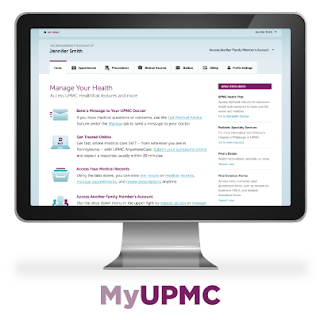The image is a left-to-right horizontal shot of a tablet or computer screen, set against a featureless white backdrop, likely the white of a computer screen. The device appears to be attached to a gray base, serving as its stand. The edges of the screen are framed in black. At the bottom of the screen, in bold purple letters, is the text "my UPMC," with "UPMC" being particularly vibrant and prominent.

In the upper left corner of the screen, there is a black mark or icon with adjacent purple text, although the exact words are indiscernible. The upper right corner of the display houses several icons, but these too are somewhat blurry and hard to identify.

On the left side of the screen, there's a black text line, possibly showing a name, potentially "Jennifer Smith." Directly opposite, on the right side, more black text can be seen, but the specifics are unclear. The interface includes various tabs at the top of the screen, with the first tab highlighted by a purple line above it. This tab reads "Manager Health" with additional black text below it.

There are multiple icons on the screen, including representations of a mail envelope, a filing cabinet, human figures, and a computer. Below the tab section, a heading in purple text is visible with additional information in black beneath it. On the right-hand side of the screen, another purple strip features more information, each section beginning with black headings followed by brief descriptions or data.